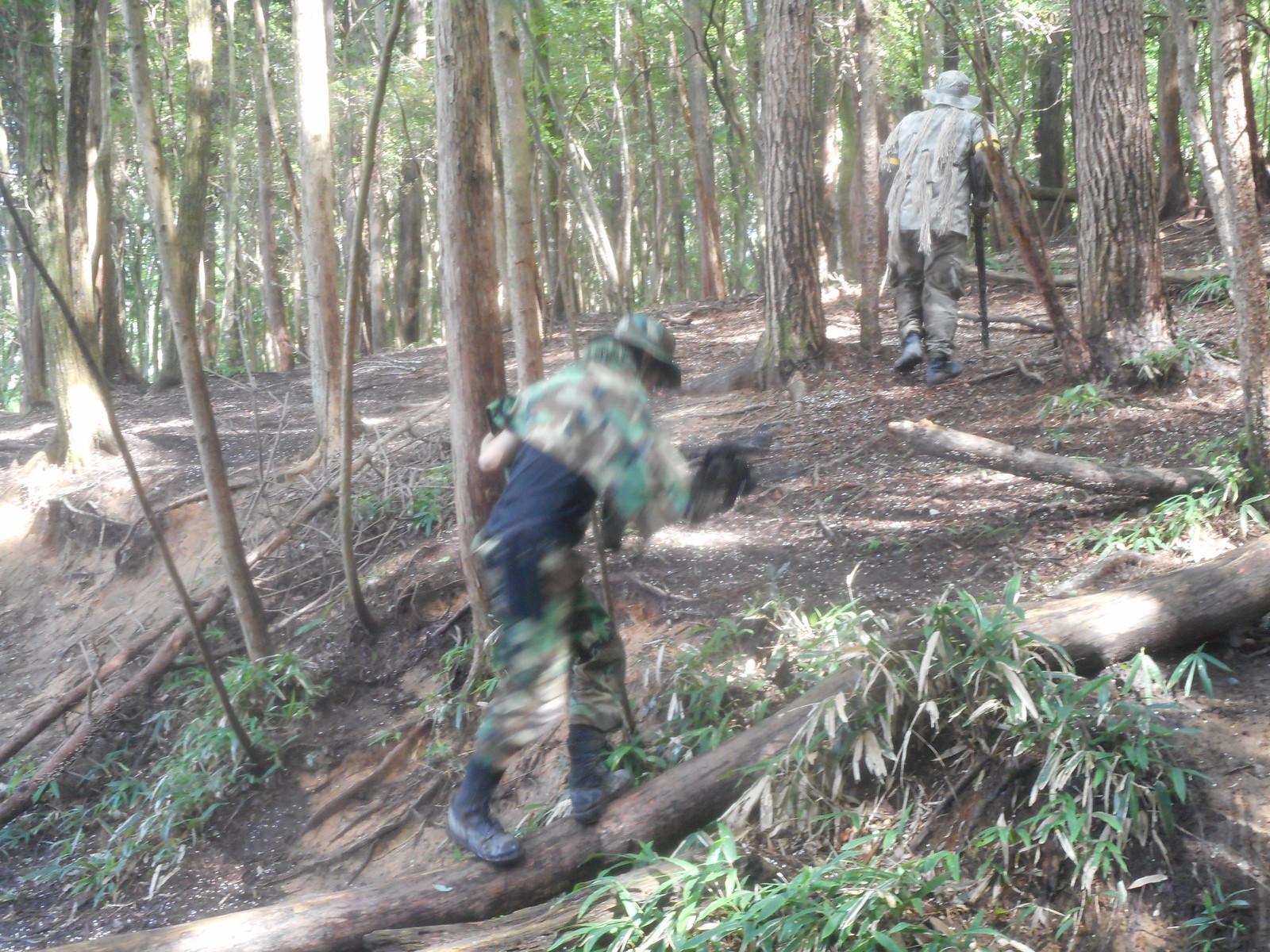The photograph captures a serene woodland scene, possibly during spring or summer, with the sun high in the sky casting a warm light over the area. The forest, characterized by clumps of green trees and sparse underbrush, features a thin log extending from a creek bed up an embankment toward a cluster of trees. 

In the image, two figures, possibly playing paintball or hunting, are dressed in varied shades of camouflage clothing, blending seamlessly with their surroundings. The figure in the foreground, possibly a child, is balancing on the log. This individual, wearing a combination of greener camouflage, a dark blue shirt, black boots, and a camouflage hat, has their back slightly turned towards the camera, creating some blurriness in the image. Further in the background, an older individual with lighter camouflage attire holds a rifle or shotgun in their right hand, appearing to lead or guide the figure on the log. The scene conveys a mix of adventure and tranquility, with the detailed attire emphasizing the purposefulness of their outdoor activity amidst the quiet and concealed beauty of the woods.